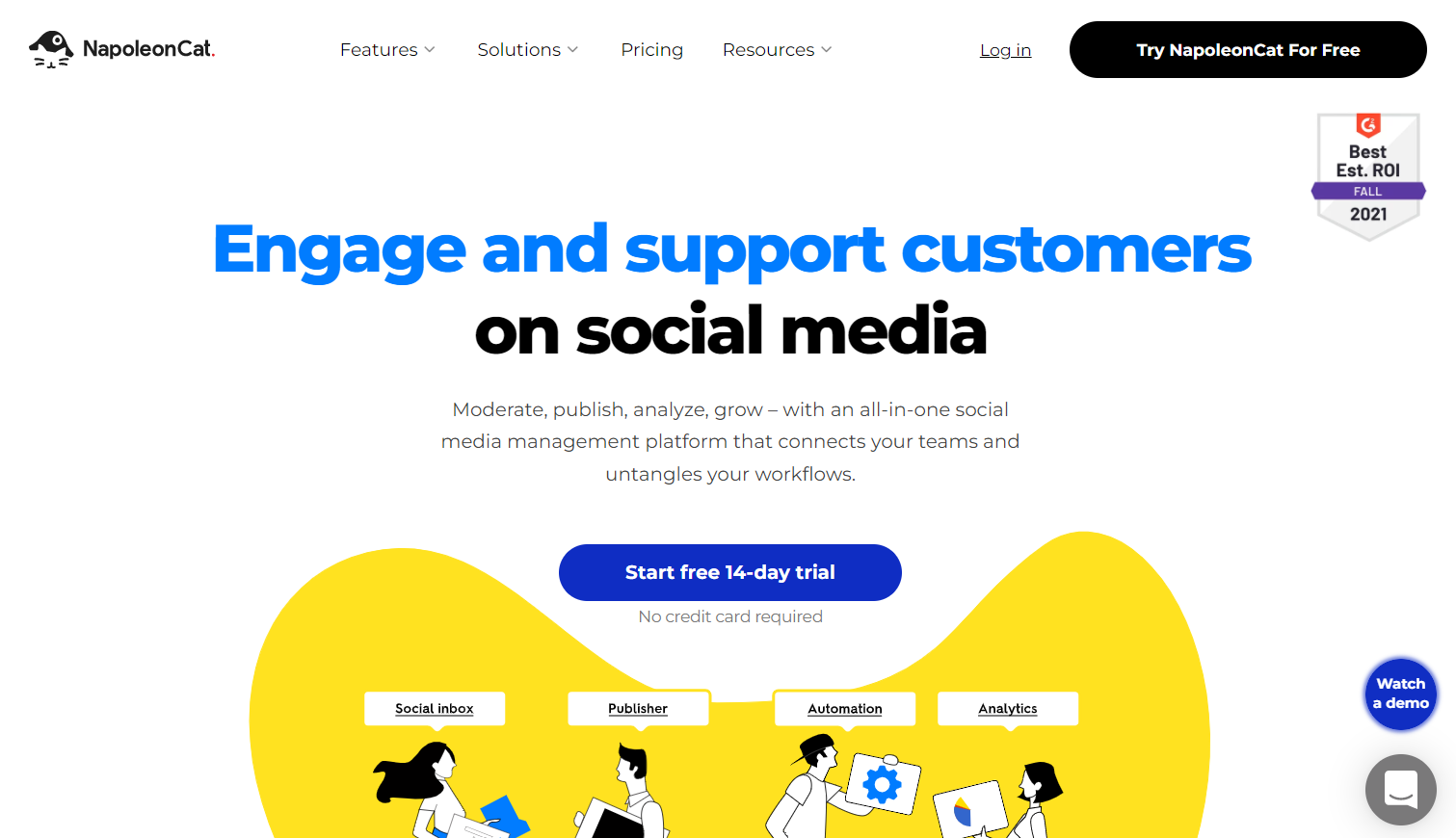The image is a screenshot of a website, prominently featuring branding and navigation elements at the top. In the upper left corner, the text "Napoleon Cat" can be seen next to the logo—a white cat silhouette with visible eyes and mouth in black, topped with a circular, black shape resembling a hat or hair. Adjacent to this are dropdown menus labeled "Features," "Solutions," and "Resources," with "Pricing" being a standalone menu without a dropdown. Further right, there is an underlined "Login" link and a black rectangular button with rounded edges, inscribed with white text that reads "Try Napoleon Cat for Free." Near this button is a "Best S-R-O-I Fall 2021" logo, depicted as a square with a triangular bottom edge.

In the center of the image, the website's main headline states, "Engage and Support Customers" in light blue, followed by a bold black subheading "Own Social Media." Below this, a smaller black text elaborates: "Moderate, Publish, Analyze, Grow, with an all-in-one social media management platform that connects your teams and untangles your workflows." Beneath this description, there is a dark blue, rectangular button with rounded edges, featuring white text that reads "Start Free 14-Day Trial."

The lower section of the image showcases a yellow bean-shaped background design with silhouettes of four people interacting, holding envelopes and posters. All individuals have black hair and white shirts, with one person sporting a black, upside-down baseball cap. Above these figures are white, square text bubbles with black text, labeled from left to right: "Social Inbox," "Publisher," "Automation," and "Analytics." In the bottom right corner, there are two circular buttons: a dark blue circle with white text that reads "Watch a Demo," and a dark gray circle featuring a text bubble with a smiley face.

The entire screenshot is set against a clean white background, creating a professional and organized appearance.